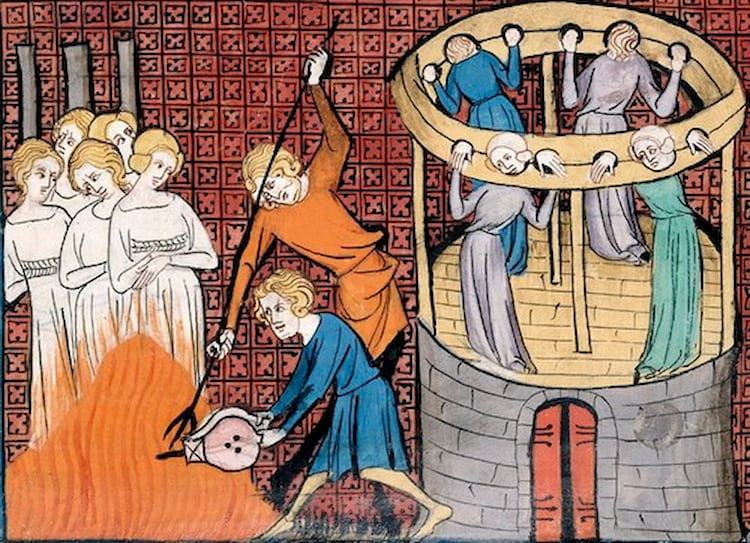The image depicts a disturbing medieval scene with a tower made of gray stone situated on the right side. Atop the tower, four individuals are held captive, their heads and hands locked in wooden stocks, preventing movement. The tower, detailed with an orange door featuring horizontal black lines, looms over the activity below. On the ground to the left, two men tend to a fire; one man, donned in a blue robe, uses a bellows to fan the flames, while the other, wearing an orange robe, wields a pitchfork with a forked end. Both appear focused on the fire, which intensifies the grim atmosphere. Standing further to the left, a group of five women, all with blonde hair styled at the back of their necks, wear matching white gowns with wide necklines. They stand in a line, hands folded at their waists, intently observing the scene. The background features a repetitive pattern of red squares marked with black Xs, adding to the eerie and oppressive feeling of the artwork.